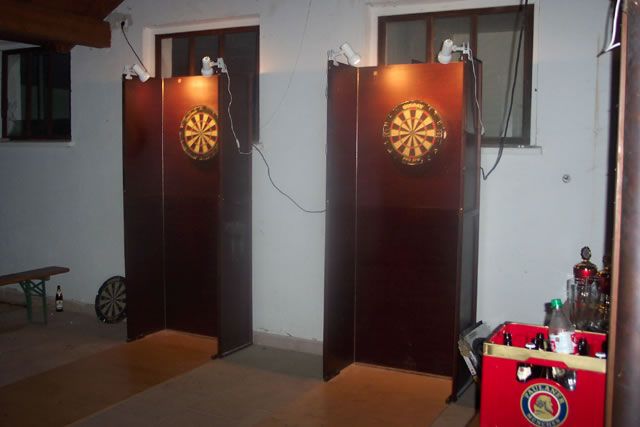The image depicts a basement room or possibly an establishment, characterized by its high-up windows, indicative of a basement setting. The room prominently features dartboard setups, composed of two freestanding trifold screens made of brown wood, each approximately six feet tall. Each screen has a wide back and narrower sides, with dartboards attached at the center. These dartboards have light tan and orange segments. Affixed to the narrow sides of each screen are white clip-on lamps, angled to illuminate the dartboards.

One additional dartboard is seen leaning against a white wall on the side. In the background, there is a low bench resembling a weightlifting bench. The room's right corner houses a red crate, likely filled with beer bottles, possibly Sam Adams, though the label isn't clear. Adjacent to this is a table or sideboard with various liquor bottles and glasses. The walls of the room are light gray, and a couple of small windows, possibly a light overhead, contribute to the lighting. Scattered around the room is a beer bottle and a red toy crate cooler with assorted drinks.